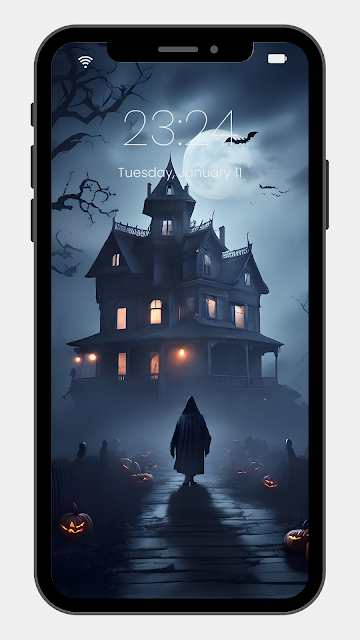The image depicts a modern smartphone positioned face up on a white surface, clearly showcasing its vivid screen. At the top left corner of the display, the Wi-Fi icon is visible, while the battery icon, indicating a full charge, is located at the top right corner. The screen wallpaper features a dark, atmospheric illustration of a tall Victorian-style house illuminated by numerous lights, including the porch lights. 

The scene is set under a full moon partially obscured by clouds on its right side, with several bats flying nearby. The time and date, "23:24, Tuesday, January 11th," are displayed prominently above the moon. In the foreground, a hooded figure is seen walking along a pathway towards the house, casting a long shadow behind them. The surrounding landscape includes bare tree branches in the upper left corner and glowing jack-o-lanterns on both sides of the pathway. A misty area is visible ahead of the figure, adding to the eerie, mysterious ambiance of the image.